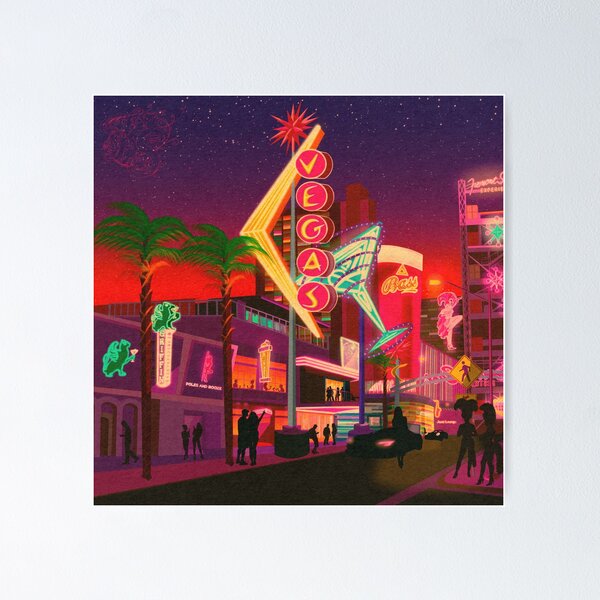This stylized, animated scene portrays a vibrant night on the iconic Vegas Strip. Dominating the center of the illustration is a large neon sign reading "Vegas" in bold letters, glowing prominently and flanked by a tipped margarita glass on one side. Along the street, palm trees with green fronds line the sidewalks, which are populated by varied silhouettes of people—some pointing at the sky, others socializing and wandering through the lively atmosphere. The scene also features various cars parked near the storefronts, enhancing the bustling urban vibe. Additional neon signs and storefronts stretch into the background, with one notably displaying "Base" and another featuring a vertically oriented sign with yellow letters on red circles and a yellow arrowhead pointing left, adding to the dazzling display. The star-filled night sky contrasts beautifully with the bright, colorful neon lights, creating a mesmerizing and iconic Las Vegas street scene.